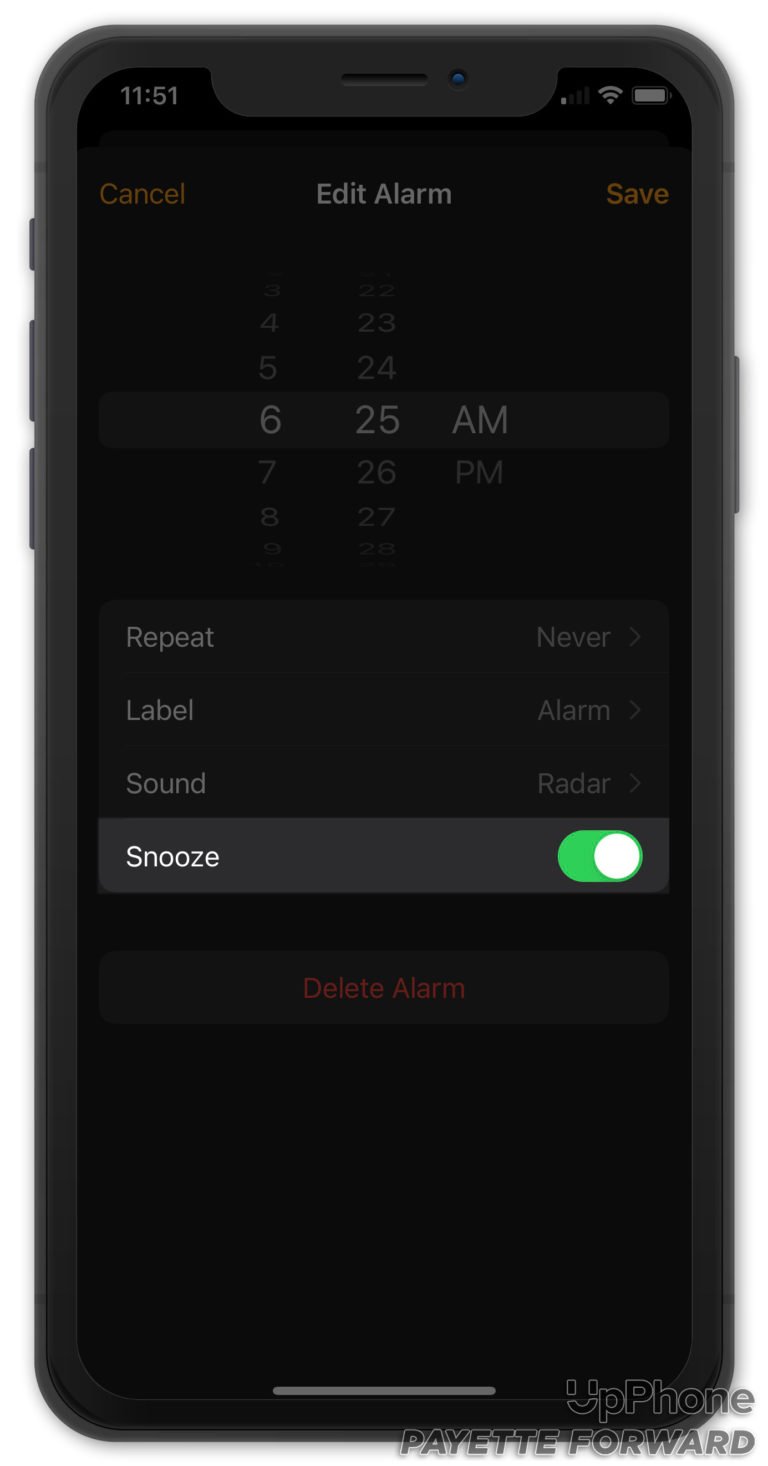A screenshot of an Android phone displayed within a black OtterBox case features a dark background and a time of 11:51 shown at the top left corner. The top right corner indicates full Wi-Fi signal strength and a fully charged battery. Below these indicators, the interface shows options related to editing an alarm. Specifically, on the left it says "Cancel", in the middle it says "Edit Alarm", and on the right it says "Save."

The set alarm time of 6:25 AM is displayed prominently, with a dial interface that allows adjustment. Under this, there are options for "Repeat", "Label", "Sound", and "Snooze". The "Snooze" option stands out in a slightly different shade of black, with a green toggle switch indicating that snooze is enabled.

At the bottom of the screen, a red rectangle displaying "Delete Alarm" is visible, contrasting with the white and gray text of other options. A fine silver bar is present at the very bottom of the screen, and a copyright notice on the right side, which appears to say "up phone pay it forward", further authenticates the image.